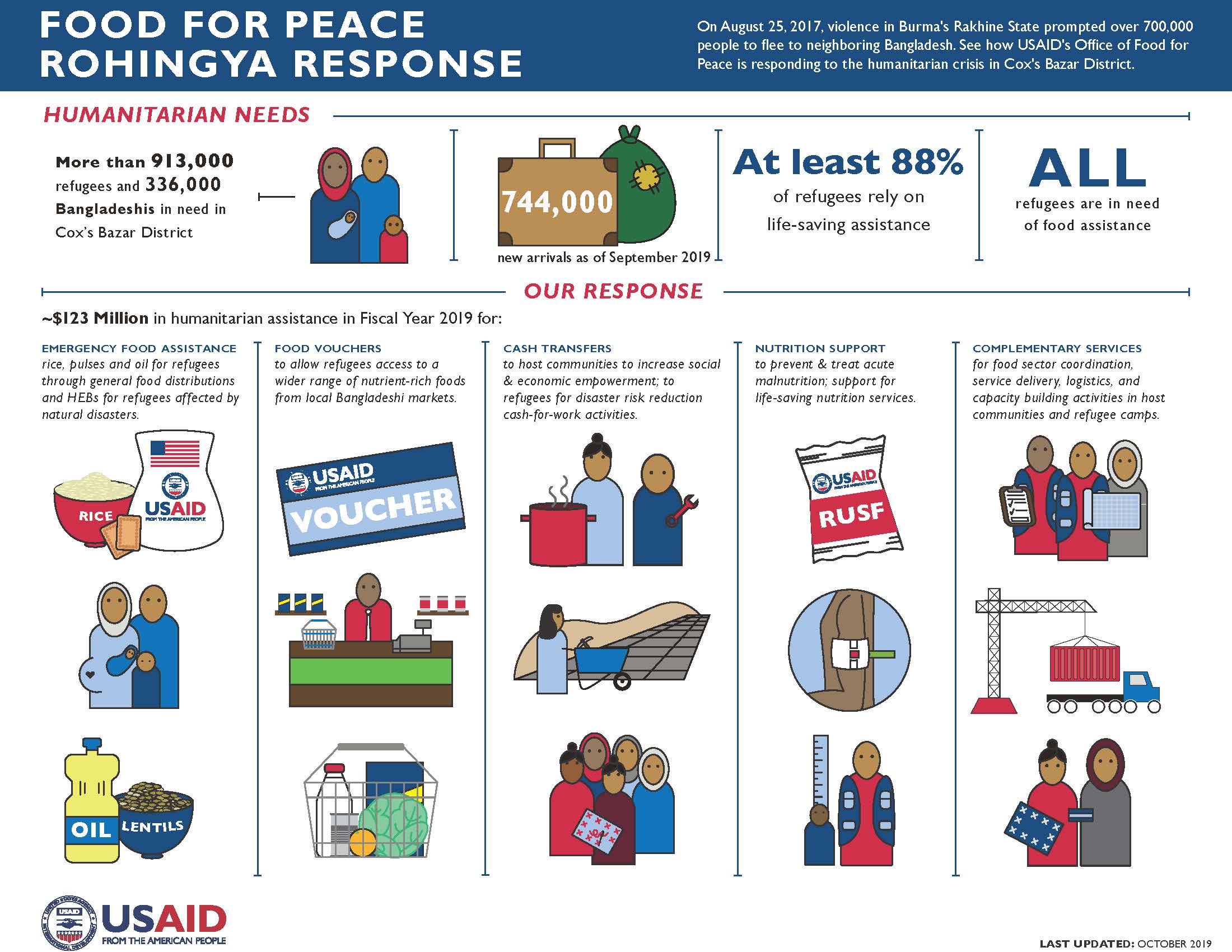This informational card or poster prominently features details about a humanitarian effort focused on the Rohingya crisis. At the top, a blue border showcases the title "Food for Peace Rohingya Response" in large white capital letters, with a brief description on the right detailing the origin of the crisis: "On August 25, 2017, violence in Burma's Rakhine State prompted over 700,000 people to flee to neighboring Bangladesh. See how USAID's Office of Food for Peace is responding to the humanitarian crisis in Cox's Bazaar District."

Directly below, the poster highlights the urgent "Humanitarian Needs" with a red header followed by significant statistics:
- A family photo depicts displaced individuals with more than "913,000 refugees and 336,000 Bangladeshis in need" in the Cox’s Bazaar District.
- Illustrated next to the family image, a briefcase icon displays "744,000" and a green bag signifies additional support.
- A crucial statistic notes "At least 88% of refugees rely on life-saving assistance," and emphasizes, "All refugees are in need of food assistance."

Further down, the card is divided into specific response sections under a heading marked in red, "Our Response," featuring five detailed columns each demarcated by thin blue vertical lines and accompanied by colorful illustrations:
1. **Emergency Food Assistance**: Rice, pulses, and oil distributions, and HEBS for natural disaster-affected refugees.
2. **Food Vouchers**: Allowing refugees access to a wider range of nutrient-rich foods from local Bangladeshi markets.
3. **Cash Transfers**: Increasing social and economic empowerment for host communities, with disaster risk reduction cash-for-work activities.
4. **Nutrition Support**: Preventing and treating acute malnutrition with life-saving nutrition services.
5. **Complementary Services**: Coordinating food sector activities, logistics, and capacity building in both host communities and refugee camps.

At the bottom left corner is the emblem "U.S. Aid from the American People," with a small, unreadable blue text beneath it, and on the bottom right, it mentions "Last updated October 2019." The poster is filled with various small, vibrant pictures depicting humanitarian assistance activities such as a bowl of rice, a family, an oil container with a bowl of beans, and other efforts showing distributions, cooking, and logistics involved in the assistance provided.

This detailed layout not only presents the scale of the crisis but also emphasizes the multifaceted response efforts and the critical support being provided to those in desperate need.